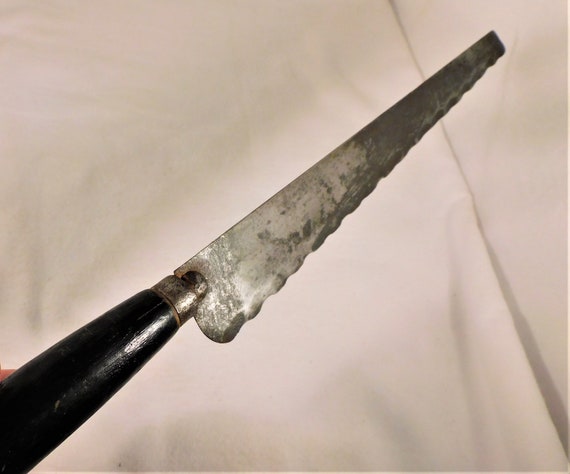The image shows an antique knife or tool with a black polished wooden handle, positioned diagonally, pointing from the lower left to the upper right. The blade is longer than the handle and tapers slightly, ending in a blunted, straight edge rather than a pointed tip. The knife blade itself is heavily tarnished with a two-tone appearance, darker near the tip, suggesting significant age and use. The cutting edge is serrated but not sharply jagged; it undulates irregularly, indicating wear or a handcrafted nature. The white background, possibly made of cloth or napkin, has discernible seams or folds, and a faint line of dust at some parts. A light-skinned finger is partially visible holding the knife at the handle.